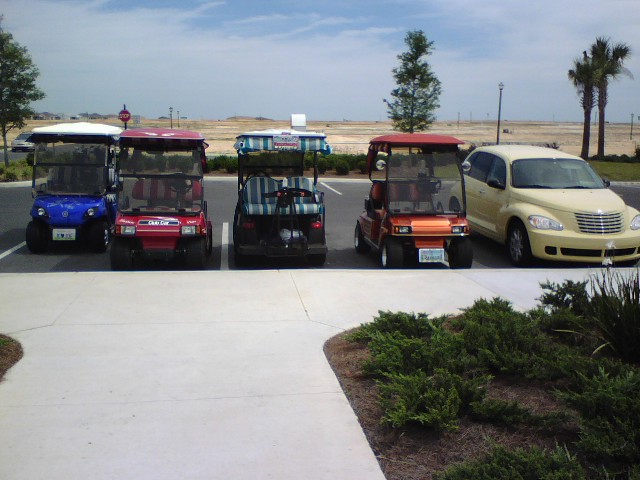This horizontal rectangular color photograph captures a parking lot scene with vibrant details. In the foreground, a broad sidewalk tees off into another, bordered by lush, landscaped shrubbery featuring blooming irises and mulched low junipers. Bright green foliage and palm trees dot the distant background, suggesting an arid, possibly southwestern U.S. environment. A flat, sand-colored expanse stretches towards the horizon, enclosed by a chain-link fence adorned with shrubs.

Dominating the scene, four assorted battery-powered vehicles in the shape of golf carts are parked beside a classic, light-cream Plymouth automobile with a silver grille. The golf carts, each with an open design and variably-screened sides, flaunt vivid color schemes: one is bright blue with a white license plate and roof; the next is entirely red with striped red and white seating; another showcases a green, blue, and white striped theme; and the fourth, bronze-colored, sits with less distinguishable interior details.

Adjacent to these, a smaller electric vehicle with a blue hood, headlights, and a contrasting deep grayish interior catches the eye. The orderly parking lines mark the pavement, and a sidewalk curb runs from the mid-left to the right side. Above, a blue sky filled with clouds enhances the framed greenery, punctuated by a stop sign indicating the structured order of this vivid, picturesque setting.